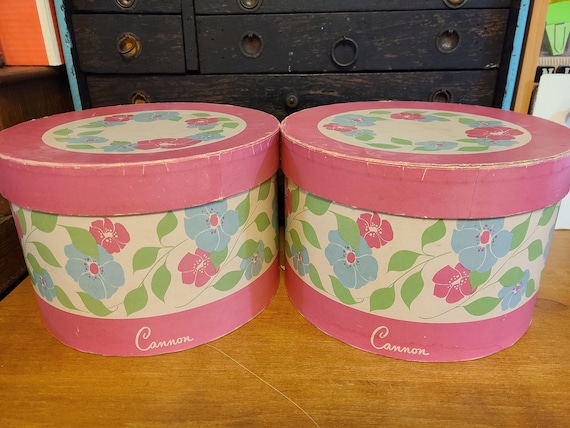This is a color photograph featuring two cylindrical boxes made of cardboard, both placed side by side on a light brownish-yellow, textured wooden table. In the background, there is a dark brown, old-looking wooden dresser, with its paint peeling and drawers fitted with unique knocker-style handles.

The two containers are identical in design and adornment, resembling decorative hat boxes or cheese boxes. Each box has a pink lid adorned with a circular floral pattern consisting of blue and pink flowers, as well as green leaves intertwined on a tan colored background. The same floral design continues along the sides of the containers, creating a charming and uniform look. At the very bottom of each box, a pink strip encircles the base, bearing the word "Canon" in white cursive script, adding a delicate finishing touch.

Overall, this image captures the vintage aesthetic gracefully, combining the worn charm of the dresser with the delicate floral accents on the cylindrical boxes.